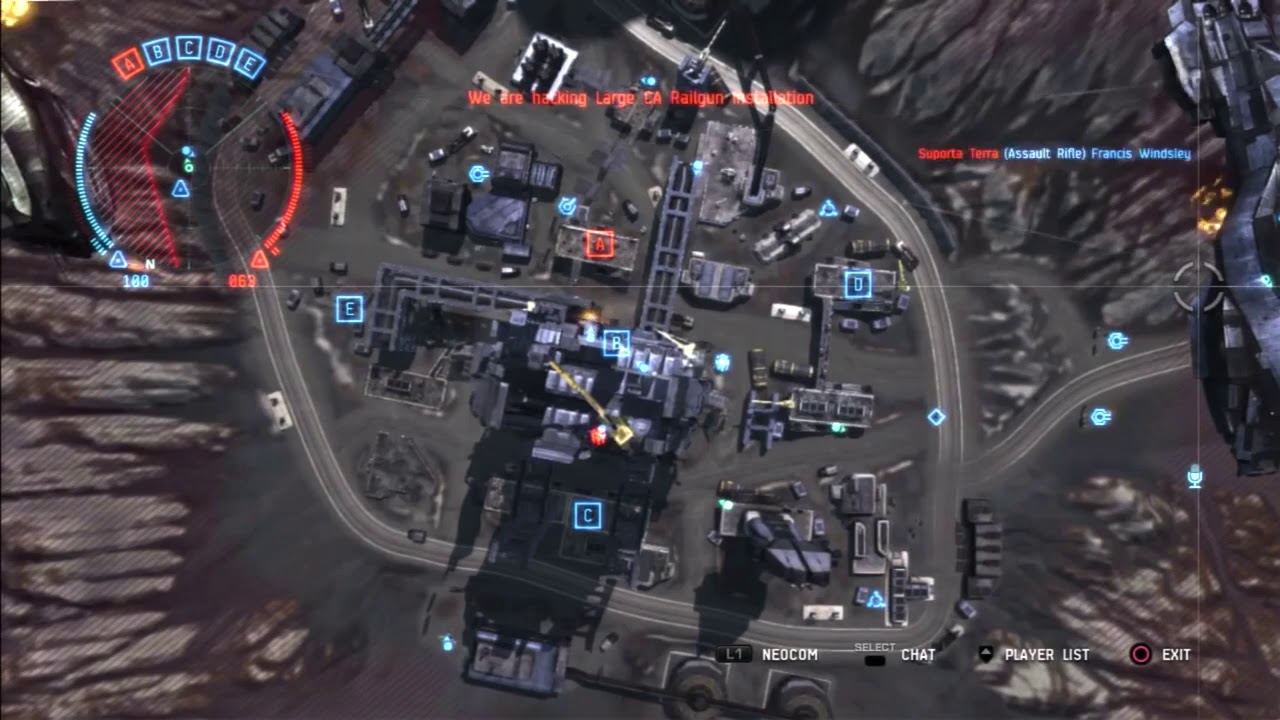This screenshot from a video game presents an overhead view of a military installation, as if viewed from a helicopter high above. The scene is predominantly dark gray, with a few red and blue highlights. It appears you are gazing into a cavern-like area encircled by rocky walls. At the center is a complex of black and gray buildings, interspersed with vehicles, possibly cars, and surrounded by a paved cement area. Circling this central area are lettered targets labeled A, B, C, D, and E, marked in blue and set inside squares. The upper part of the image features red text, partially readable as "we are...," along with the terms "large railgun" and "Assault Rifle" in blue. The bottom right corner of the screen displays game controls including "neocom," "chat," "player list," and "exit." This structured layout suggests a strategic and possibly combat-focused setting within the game.